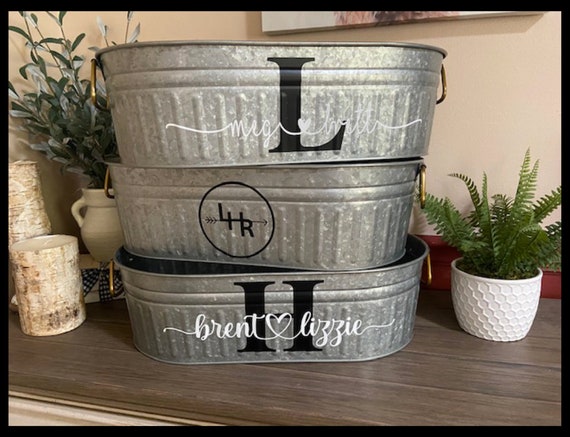The photograph captures a beautifully arranged wedding-themed decoration setup in a cozy home interior. At the center of the image, three oval, silver metal containers are neatly stacked on top of each other, each adorned with various wedding-related inscriptions. The top tub features a prominent black capital letter "L" with delicate white script reading "Meg Hart Britt". The middle tub has a black circle with a white number "4", an "R", and a horizontal arrow pointing to the right within the circle. The bottom tub displays a large black capital "H" and the names "Brent" and "Lizzie" in white script, separated by a heart symbol.

These containers are placed on a wooden surface with a noticeable grain pattern, resembling either a table or a shelf. To the right of this arrangement sits a white vase with a fern plant in a honeycomb-patterned pot, adding a touch of greenery to the setup. On the left side, there are two candles encased in birchwood bark, accompanied by another white vase holding sage leaves.

The background features a beige-colored wall with a picture hanging above the tubs, creating a warm, inviting atmosphere. This elegant display, likely set up to celebrate an upcoming wedding, exudes charm and attention to detail, showcasing the couple's names and a variety of personal touches.